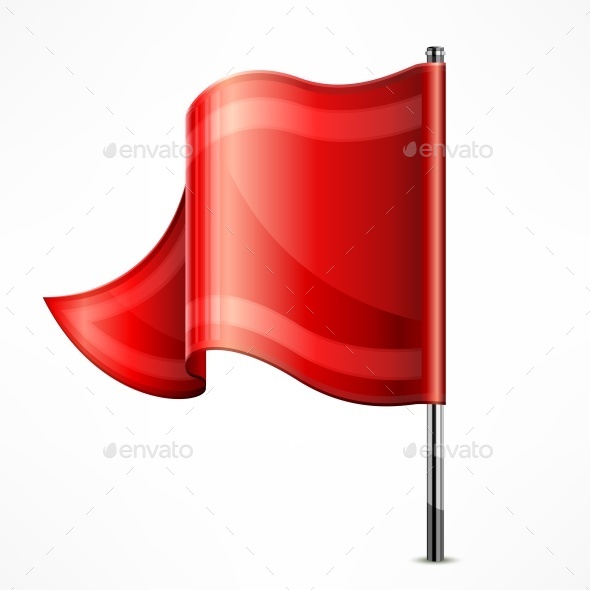The image depicts a red flag attached to a sleek, two-tone silver and gray metal pole. The flag, which flows to the left as if caught in the wind, showcases various shades of red, including lighter red tones and darker, pinkish hues. It features a lighter red rectangular border that lines the top, bottom, and edge, giving it a framed appearance. A semicircular detail emerges near the bottom and arcs toward the top of the flag. Diagonal, dotted lines span across the image, conveying a "cut here" effect. Additionally, the word "Envato" and its corresponding symbol are repeated multiple times throughout the picture.